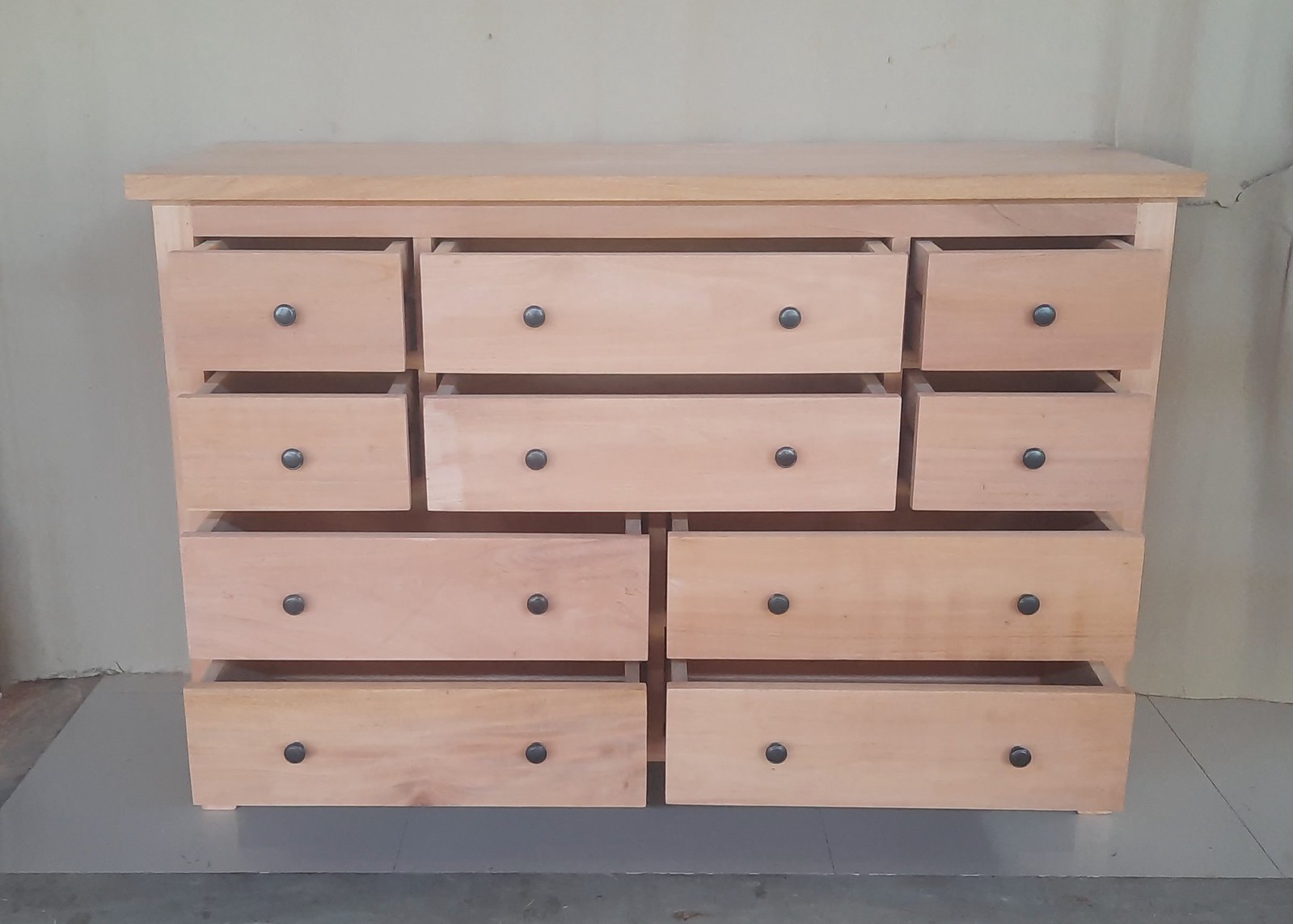The image is a color photograph taken indoors, showcasing a neatly organized light brown chest of drawers against a light green wall. The flooring appears to be covered by a grey metallic, acrylic-like floor protector. The dresser, with a flat finished top that extends slightly beyond its base, is constructed from a very pale, finely grained wood, resembling birch or maple.

The chest features four rows of drawers, all slightly pulled open, revealing their empty interiors. The top two rows comprise three drawers each, with smaller rectangular drawers on the left and right sides, and a longer, rectangular drawer in the center. Each of these longer drawers is equipped with two simple, round, dark silver or black knobs, while the smaller side drawers have a single matching knob. The bottom two rows each hold identical, longer rectangular drawers, all with two knobs. The entire dresser has clean lines and an uncluttered appearance, accentuated by the absence of any objects on its flat top. 

In the background, a white curtain-like backdrop partially frames the scene, adding a subtle contrast to the dresser's minimalist design.